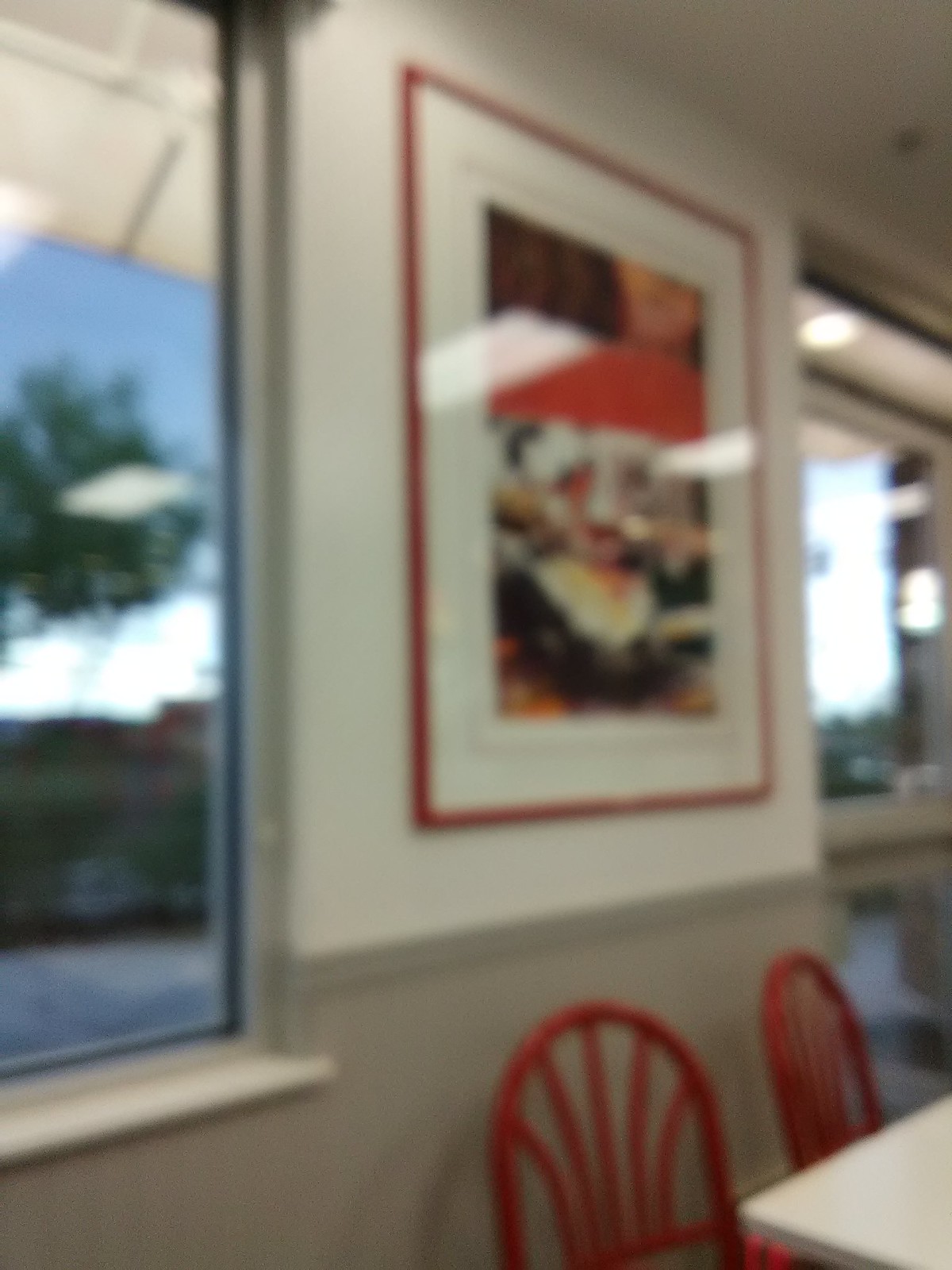This image captures a slightly blurry interior of a restaurant featuring a cozy, albeit unclear, ambiance. Against the backdrop of white and khaki two-toned walls, two red chairs are snugly positioned against a wall, partially revealing a table’s corner. On the left side, a window opens up to a wintry, almost-dark outdoor setting, suggesting the cold and the approaching evening. To the right of this window, a striking large piece of art hangs prominently on the wall, enclosed in a bold red frame with a white matte. The artwork within, vivid with hues of red and black, intriguingly showcases a design that appears to include a teddy bear or panda bear. Further to the right, partially visible deeper into the restaurant, is a second window. The combination of these elements hints at a warm, inviting space that contrasts with the chilly exterior, creating a detailed and textured visual narrative despite the photograph's lack of clarity.